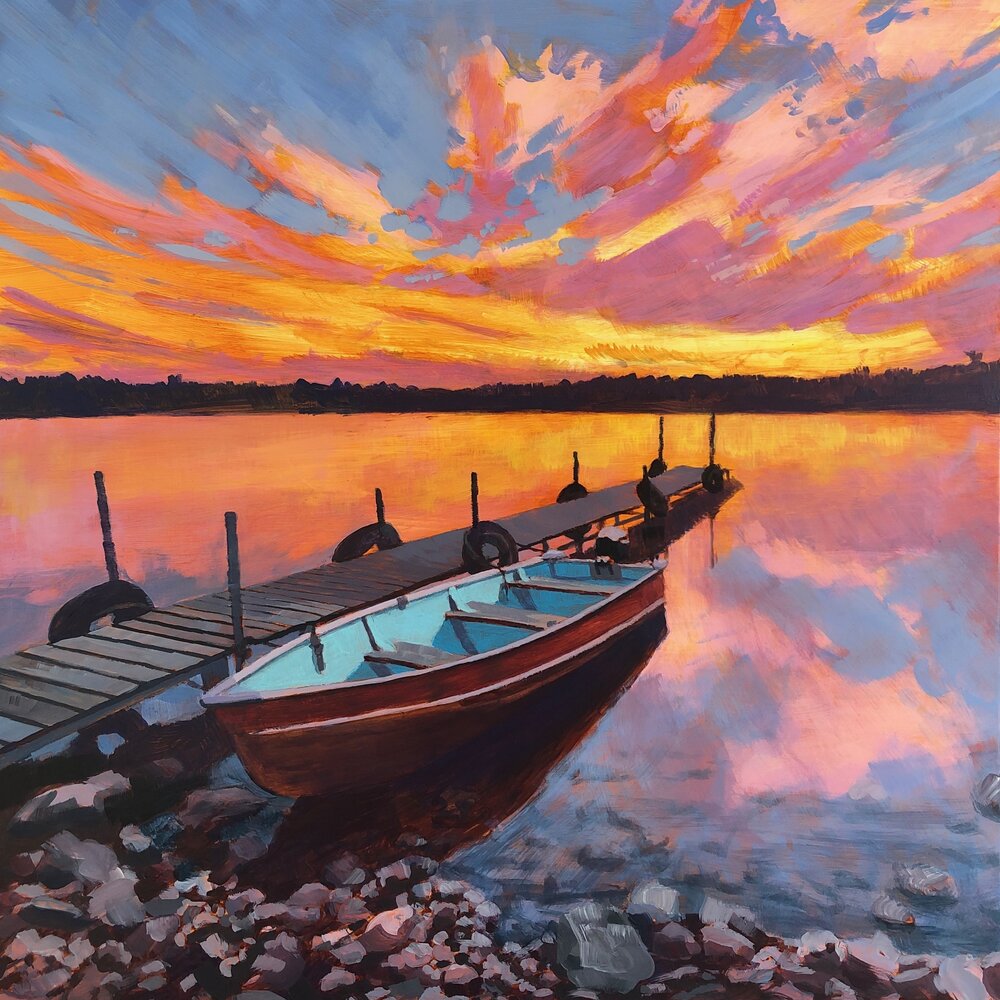The painting, a stunningly realistic color artwork, depicts a serene lakeside scene at sunset. The square-format image measures approximately six inches by six inches, capturing a tranquil moment with meticulous detail. The upper portion of the painting features a sky painted in beautiful hues of orange, pink, yellow, purple, and blue, with swooping clouds scattered towards the top, giving way to a clear blue-gray sky. The horizon showcases a silhouetted row of trees and hills, rendered in dark, almost black tones due to the approaching dusk.

Below the horizon, the lake's still waters mirror the vibrant colors of the sky, creating a seamless transition from the heavens to the earth. A long wooden pier, extending about 70 to 80 feet from the left foreground towards the center, juts into the lake. The pier, made of horizontal gray wood and adorned with black tires as bumpers along its vertical posts, enhances the rustic charm of the scene.

Prominently featured is a shallow, open fishing boat docked to the right side of the pier. The boat, painted in a distinctive reddish-brown with a white stripe along its side, has a blue interior with three or four wooden plank seats and a small outboard motor mounted at the back. Positioned with its bow facing the bottom left corner of the image, the boat suggests readiness for a tranquil outing. Surrounding the pier and boat, the shoreline is detailed with brown pebbles and rocks, adding texture to the foreground.

Overall, the painting masterfully blends the reflective calm of the lake with the warm, descending light of the sunset, offering a captivating and serene outdoor scene.